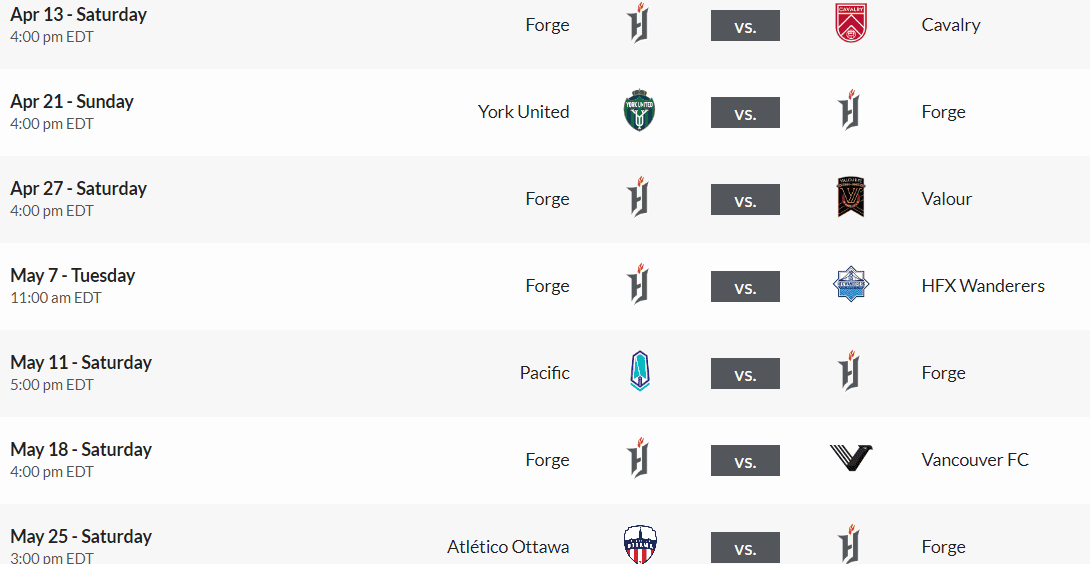This image showcases a detailed football timetable for various matches. The schedule is laid out in a clean, reader-friendly format with alternating light gray and white backgrounds for each row to enhance legibility. Each match listing includes the date, day, and time in EDT (Eastern Daylight Time) along with the teams' names and logos, separated by a gray "versus" box. The entire schedule suggests that the matches are based in Canada, with teams such as Ottawa, Vancouver, and other Canadian cities featured prominently.

1. **April 13th, Saturday, 4 p.m. EDT**: Forge vs. Cavalry
2. **April 21st, Sunday, 4 p.m. EDT**: York United vs. Forge
3. **April 27th, Saturday, 4 p.m. EDT**: Forge vs. Valor
4. **May 7th, Tuesday, 11 a.m. EDT**: Forge vs. HFX Wanderers
5. **May 11th, Saturday, 5 p.m. EDT**: Pacific vs. Forge
6. **May 18th, Saturday, 4 p.m. EDT**: Forge vs. Vancouver FC
7. **May 25th, Saturday, 3 p.m. EDT**: Atlético Ottawa vs. Forge

The timetable excludes any additional information beyond the match schedule, focusing purely on the upcoming football matches.